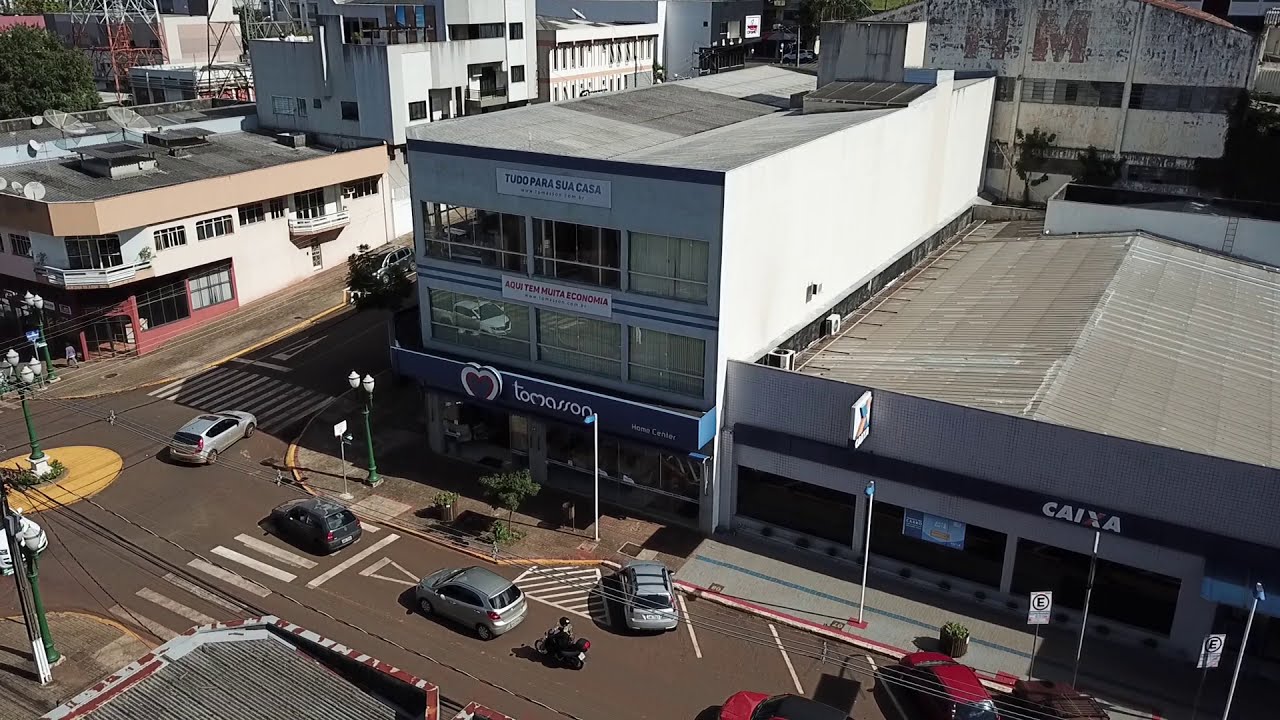The aerial view image captures a bustling urban setting characterized by multiple businesses. Central to the scene is a prominent three-story building housing several establishments, with the ground floor business named Tomasin, identifiable by its distinctive blue sign adorned with a red and white heart. Directly to the right of this building is another business branded with the letters C-A-I-X-A on its signage. The foreground reveals a busy street lined with various cars, some parked diagonally and others in motion, suggesting a lively traffic flow. In the top left of the image is a building with a red storefront contrasted against its white upper floors, adding a splash of color to the scene. To the left of the center, a large light post stands out prominently. The background shows a mix of industrial elements, including visible cranes, and older, seemingly neglected buildings, adding layers of depth and texture to the urban landscape. Additionally, there are visible crosswalks and even a roundabout, emphasizing the organized yet dynamic nature of this cityscape.